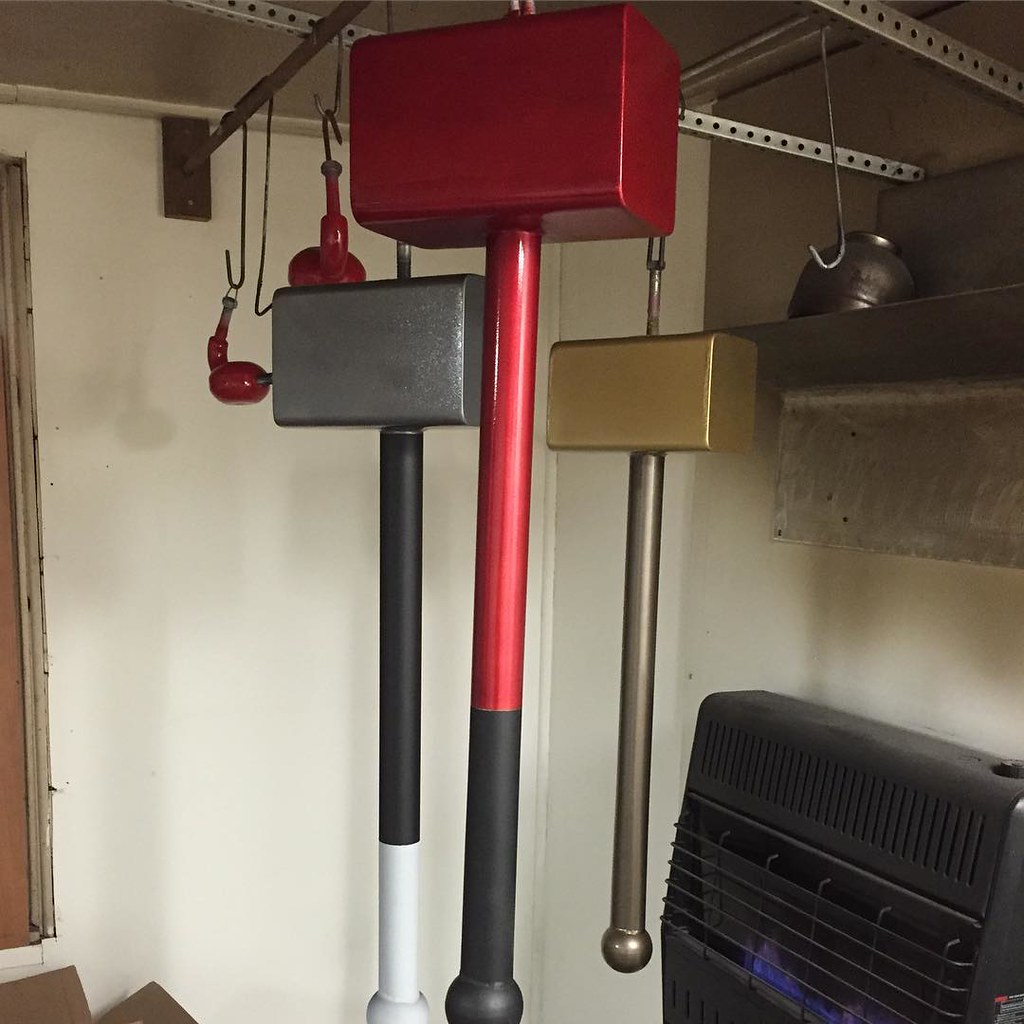The image is an indoor scene with light beige, almost off-white walls that meet a darker, gray-toned ceiling. There are rectangular metal beams, about an inch-by-inch in size, running across the upper part of the wall with small holes perforating them. These beams support hooks that hold three large sledgehammers. The sledgehammers have a novelty appearance reminiscent of comic book weapons, such as those used by Thor.

In detail, the hammer in the center features a red head and a black handle. On the left, the hammer has a gray head with a handle that is black at the top and white at the bottom. The rightmost hammer stands out with its golden head and a handle that appears to be silver. All the hammer heads are rectangular in shape.

Additionally, towards the bottom right corner of the image, there is a black item that resembles a portable heater or possibly an air conditioner, with a blue flame visible, indicating it could be a gas heater. The setting resembles a garage, with silver shelving and a small silver pot positioned midway up the wall on the right-hand side. The braces and metal structures supporting the hooks show signs of rust, adding to the garage-like ambiance.